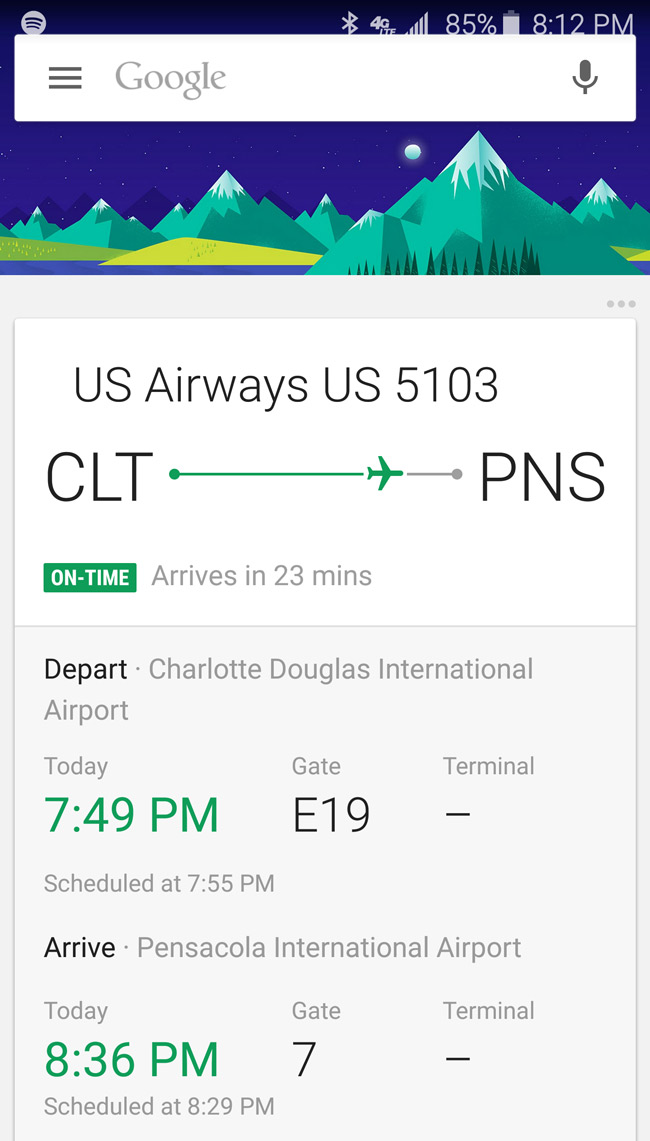The image captures a screenshot of a Google search page. Centered prominently beneath the iconic Google search bar is a scenic, digital illustration featuring a deep, royal blue sky adorned with twinkling white stars and a distant moon. This celestial backdrop contrasts beautifully with the vibrant green mountains below, some of which are capped with snow, giving a striking visual display of nature.

At the base of the mountains, clusters of trees are visible, mingling with patches of purple, white, and yellow terrain, adding depth and color to the landscape.

Superimposed on this picturesque scene is detailed flight information for U.S. Airways Flight 5103. The data reveals that the flight from Charlotte Douglas International Airport (CLT) to Pensacola International Airport (PNS) is on time, highlighted with a green status indicator. The flight is scheduled to arrive in 23 minutes.

Specific details include:
- Departure from Charlotte Douglas International Airport (CLT) today at 7:49 p.m. from Gate E19. The terminal information is absent.
- Arrival at Pensacola International Airport (PNS) is expected today at 8:36 p.m. at Gate 7, with the flight originally scheduled to land at 8:29 p.m. The terminal information is also missing for the arrival.

This detailed view offers both a tranquil scenic image and precise, real-time flight tracking information.